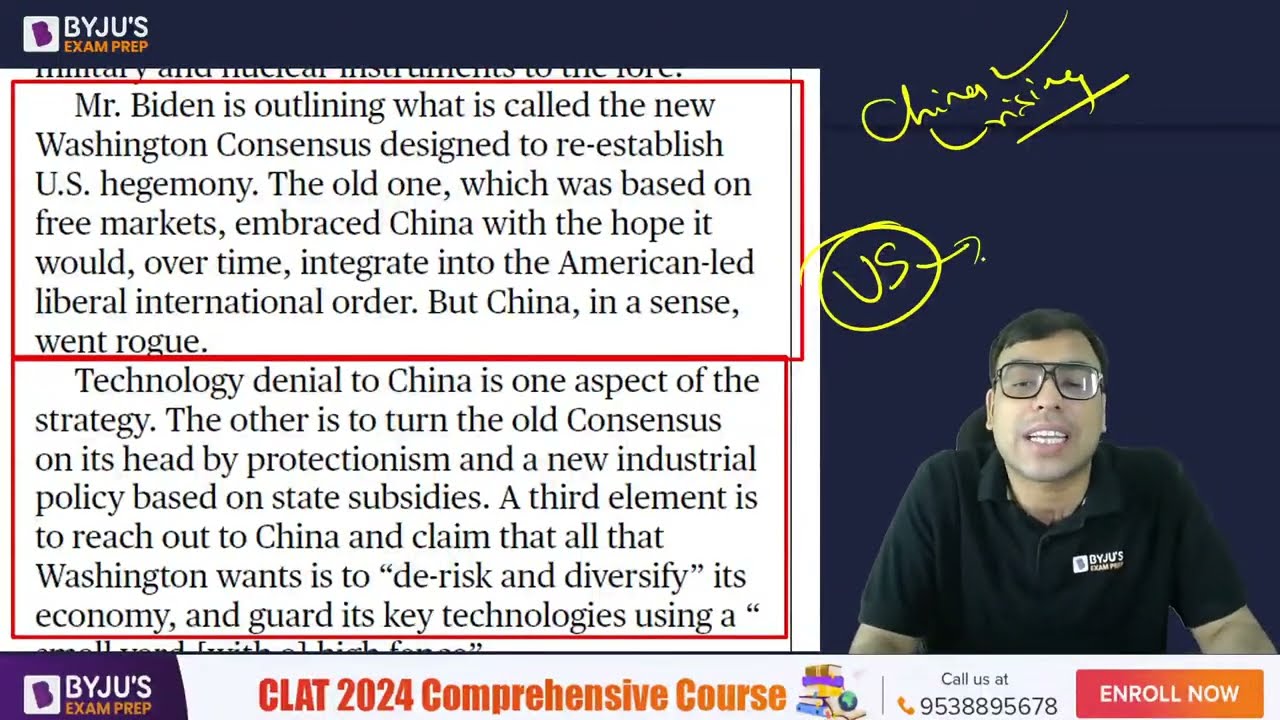The image depicts an online class video recording featuring a young male tutor, identifiable by his short black hair, glasses, and a black T-shirt emblazoned with the BYJU's logo. Located in the bottom right corner of the image, he is seated in an office chair against a background interspersed with text and graphical elements.

In the upper left corner of the image, the BYJU's Exam Prep logo is prominently displayed against a dark blue background, which continues throughout the image. On the left side of the image, there is a white rectangular section filled with printed text described as a news clip or a poster. This text references Mr. Biden outlining the "New Washington Consensus," aimed at reestablishing U.S. hegemony by reversing the old consensus based on free markets and addressing China's role within it. It mentions specific strategies such as technology denial to China, protectionism, and state subsidies, as well as efforts to de-risk and diversify the economy while guarding key technologies.

Handwritten text in yellow marker, including the words "US," "China," "rising," and "default," with some underlined and circled, is superimposed on this section, indicating the tutor's likely annotations during the lesson. The bottom central portion of the image prominently features the heading “CLAT 2024 Comprehensive Course,” accompanied by a logo of books and globes, a phone number (9538895678), and an "ENROLL NOW" button. Additional BYJU's logos appear on both the top left and bottom left corners of the image, reinforcing the branding for the online educational course.